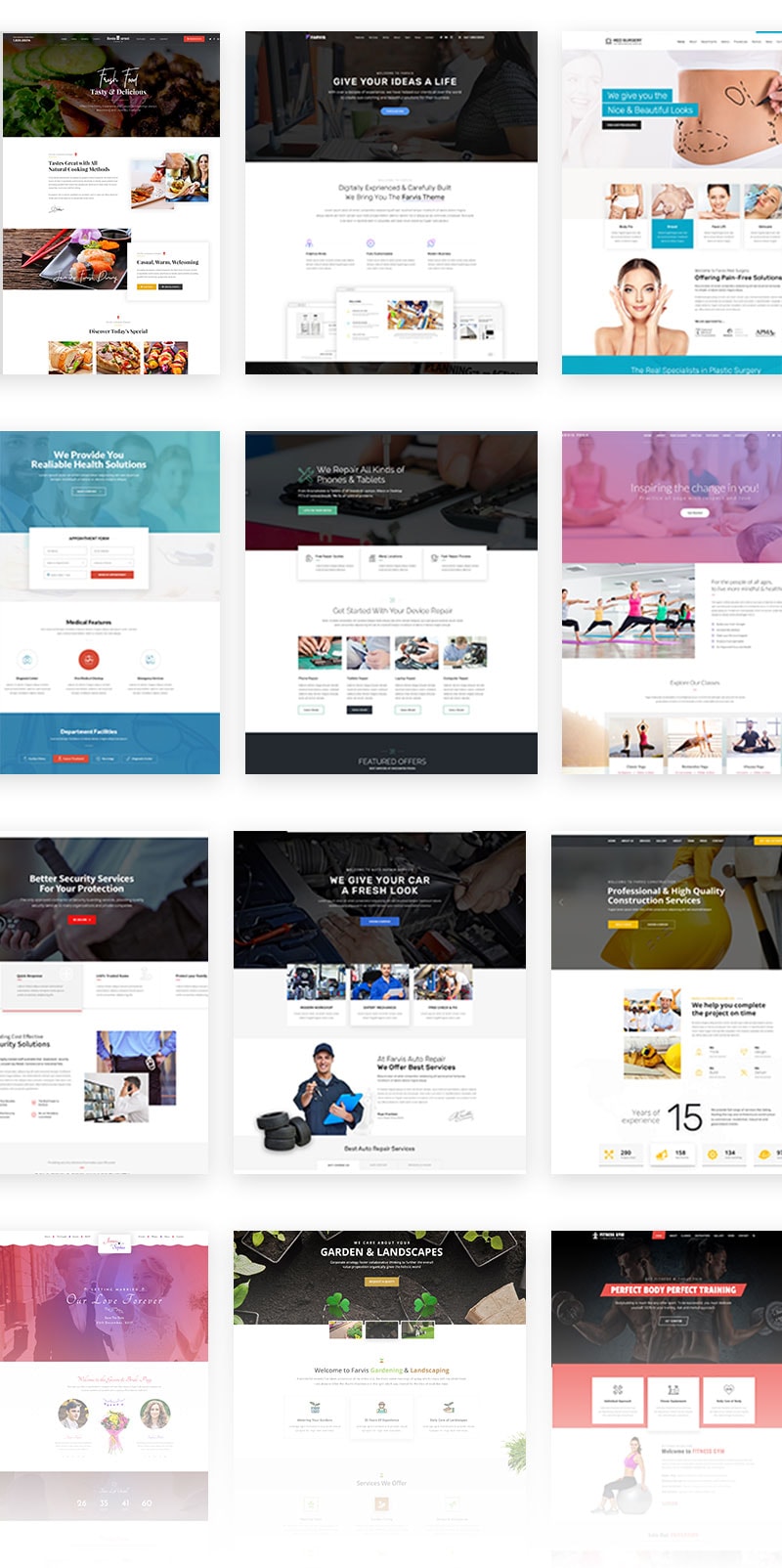The image features a light blue background with a grid arrangement of 12 smaller images, each showcasing diverse elements and details.

1. The first image has a dark background with text, a picture of people, food, and three smaller images at the bottom. It also includes a yellow box and a black box.
2. The second image also has a dark background at the top, with text and a small blue box. It features a picture at the bottom with black trim at the base.
3. The third image displays a pink cushion and four smaller pictures below it. A woman appears to be scrubbing her face, accompanied by a blue box.
4. The fourth image is blue on top with a white inset containing a red box with a red circle. The bottom portion is blue with another small red box.
5. The fifth image has a black top section with a green box and a white inset featuring four small pictures and a black box at the bottom.
6. The sixth image has a purple top with a white box, a picture of people exercising, and four more smaller pictures below.
7. The seventh image, with a dark top and a red box, contains two pictures. The bottom part also has a dark section with a blue box and three pictures, followed by a large image.
8. The eighth image features a yellow top with a small yellow box, a picture with something yellow and the number 15.
9. The ninth image has a purple background, three small pictures, and a purple bottom section.
10. The tenth image has a dark background with a white print, a yellow box, and three smaller pictures.
11. The eleventh image is dark with a pink box, followed by a larger pink box containing three small white boxes.
12. The twelfth image shows a person sitting and exercising against a dark background.

This detailed description captures the intricate layout and diversity of elements within each of the 12 smaller images featured on the light blue background.